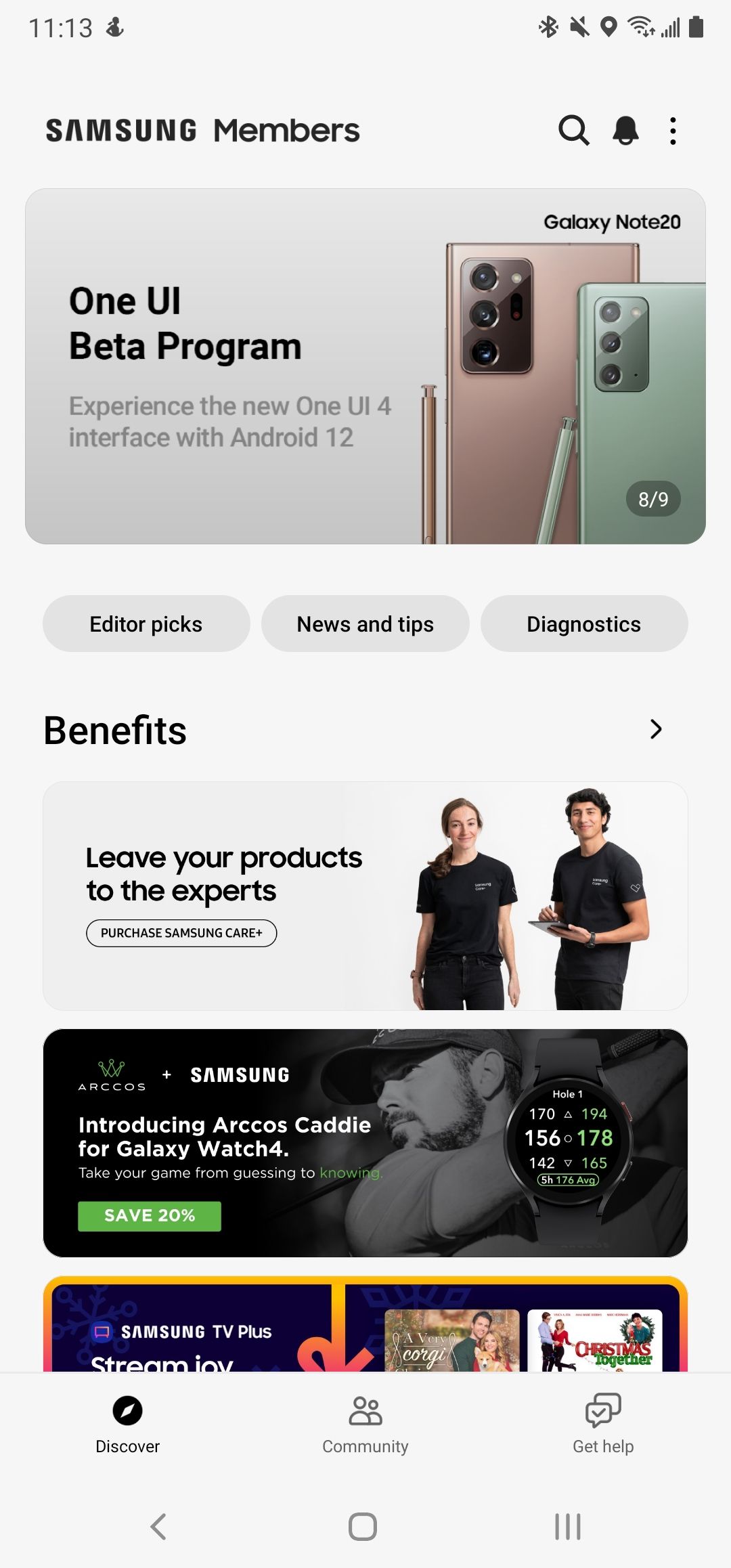**Detailed Caption:**

This is a detailed color image of a mobile-optimized website displayed on a Samsung smartphone. The background is primarily white, ensuring a clean and minimalistic look.

At the very top of the screen, aligned to the left, is the current time displayed in black text, showing 11:13. To the right are various mobile icons indicating connectivity features such as Wi-Fi.

Beneath the status bar, the page header reads "Samsung Members" in black text. This header also includes a search icon, a bell icon likely for notifications, and a menu icon represented by three vertical dots, all positioned towards the right.

Following the header, there is a distinctive darker rectangle that features an image of two Samsung Galaxy smartphones. One phone has a pink back, and the other has a green back, each accompanied by a stylus placed to its left. To the right of these phones, text partially displaying "Samsung Galaxy" and "Model 20" is visible, though the much smaller text is not entirely readable. The left side of the rectangle promotes the "One UI beta program," encouraging users to "experience the new One UI 4 interface with Android 12."

Below this promotion, three rounded grey rectangles with black text serve as buttons, labeled "Editor," "Pics," "News and Tips," and "Diagnostics."

The next section, titled "Benefits," presents an image of a man and a woman both wearing black t-shirts and black trousers. The accompanying text promotes service reliability: "Leave your products to the experts," though additional smaller text in a nearby rectangle is not legible.

Further down, a black section includes an image of what appears to be a man's head. White text reads, "Introducing Arcadius cable for Samsung Galaxy watches. Save 20%." Below this is a partially visible blue and multicolored caption or image that is cut off and unreadable.

At the very bottom of the screen, navigation buttons include "Discover," "Community," "Get Help," along with a back button, a home button, and an icon of three vertical columns, likely representing a menu or additional options.